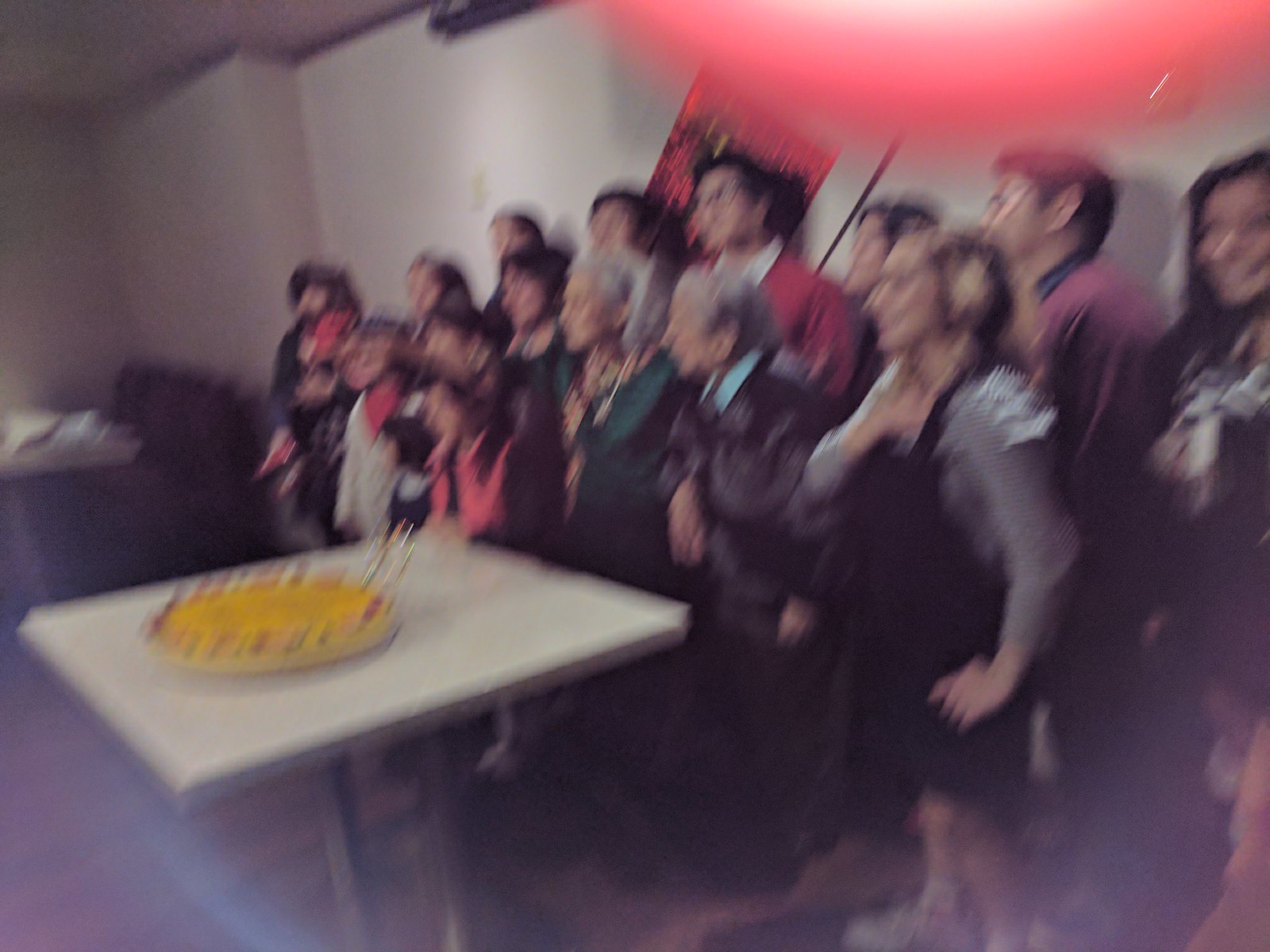This image features a very blurry photograph of a group of approximately 16 to 20 people standing in two rows in front of a white, indented wall in a large, commercial-looking room that could be a restaurant, dining room, hall, or bar. The people range in age from young adults to elderly, with a mix of men and women. The taller individuals are positioned in the back row, with many of them having dark hair, while the shorter ones are in the front row. In the center, there are two elderly people with grey hair. In front of the group is a square table with a white top and two steel legs. On the table sits a large, circular yellow cake adorned with numerous candles. To the left of the group is an out-of-focus brown leather couch. The flooring appears to be wooden. At the top right corner of the image is a reddish light source, possibly mistaken for a balloon. Though the image is quite blurry, particularly around the edges, it seems to capture a celebratory moment, possibly an elderly person's birthday party.